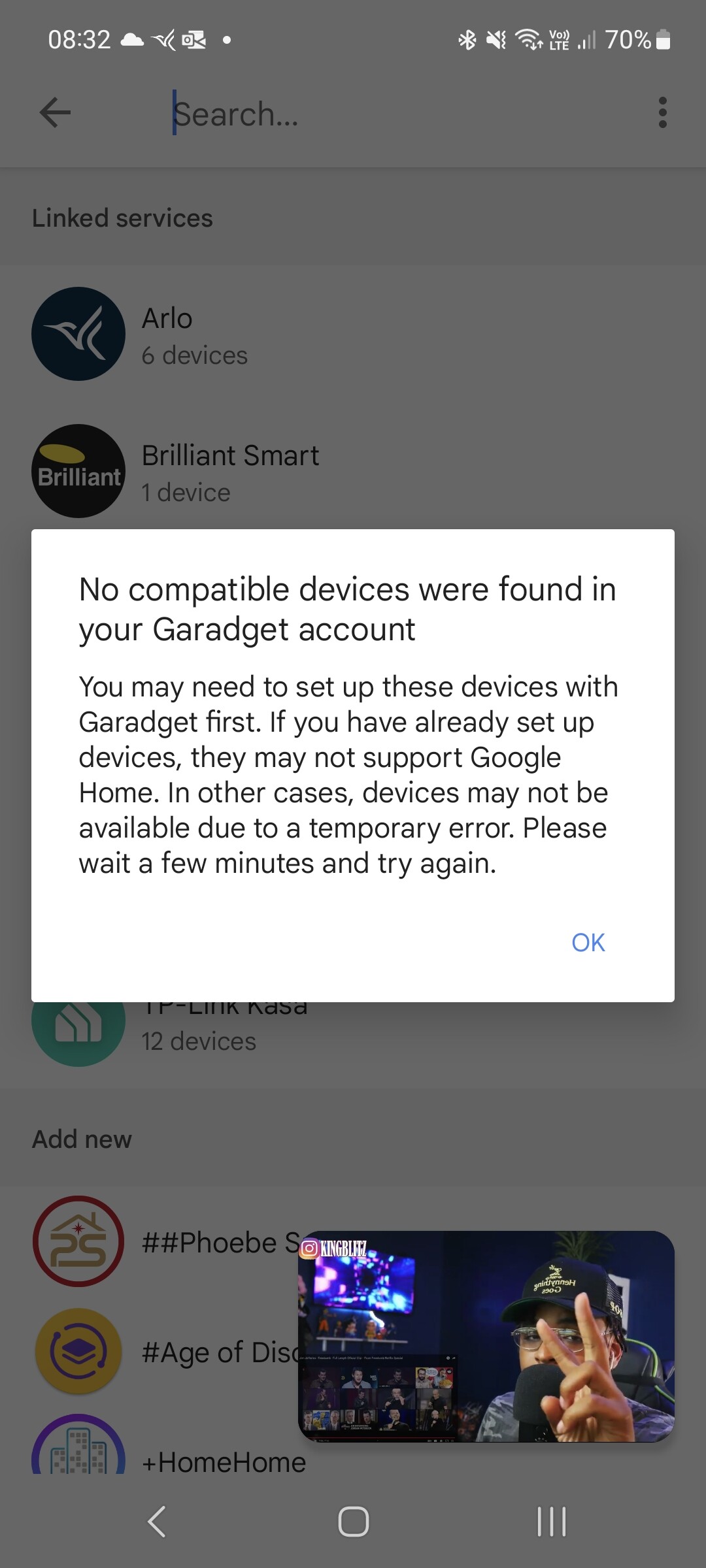The image depicts a dialogue box with a grayed-out background. At the very top of the box, a bold text message reads, "No compatible devices were found in your GarageGet account." The main body of the dialogue box contains a detailed message stating: "You may need to set up these devices with GarageGet first. If you have already set up devices, they may not support Google Home. In other cases, devices may not be available due to a temporary error. Please wait a few minutes and try again." In the lower right corner of the dialogue box, there is a blue button labeled "OK." The overall visual context suggests that the user is being informed of an issue with device compatibility or availability within their smart home system.